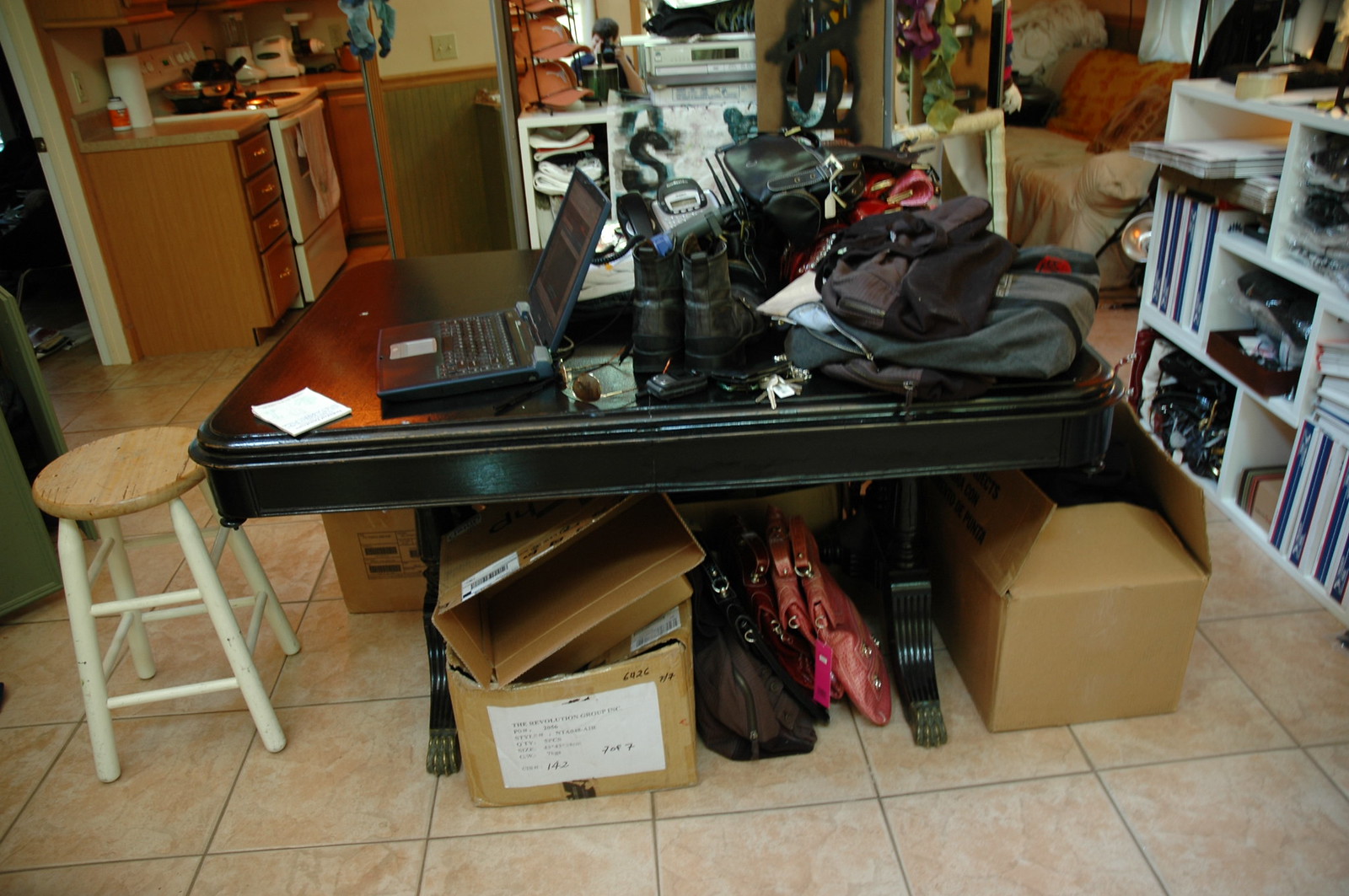This image captures the essence of a cluttered yet character-rich studio apartment. Dominating the scene is a large, ornate black dining table, which appears to be an antique painted in black. The table is laden with various items, including a computer, a laptop, a pad and paper, a cell phone, several purses and bags, and a pair of black work boots. A low, white bar stool with light wood accents serves as a chair for the table, adding a touch of modernity to the antique look.

Beneath the table, a chaotic pile features empty boxes and both black and pink book bags. To the right, a white, modern bookshelf stands out, filled with blue and white books, as well as some folders. This adds both aesthetic and functional value to the space.

In the background on the right, part of another room is visible, alongside a compact kitchen nook that includes a stove, a toaster, and some cupboards. Items like a roll of paper towels and pans on the stove clutter the countertop, emphasizing the lived-in feel of the apartment. The kitchen floor is tiled with large, terra cotta-colored beige tiles.

Further in the background, a sofa bed with an orange backrest and a beige sheet draped over the seat is visible. Adjacent to it, chrome shelves hold a stereo system and a stack of amber-colored baseball hats, blending leisure with utility. The overall scene is eclectic and busy, a true reflection of the multifaceted life of its occupant.